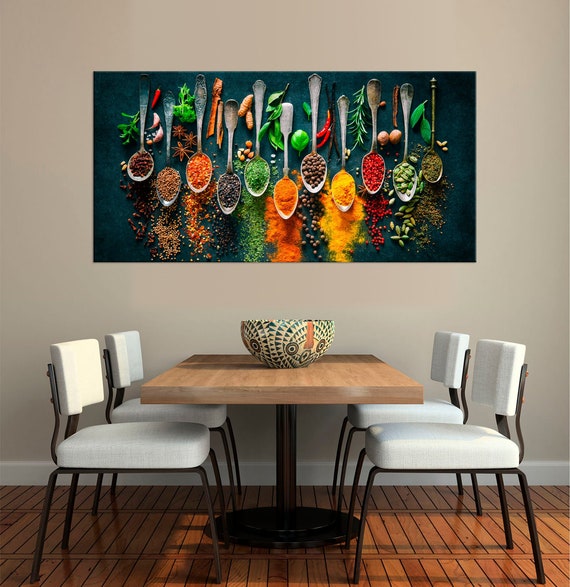The image depicts a cozy dining room with a simple, diner-style table featuring a single central pole and a light brown top. It is surrounded by four stubby chairs, each with white padding and backs, supported by stout metal legs. The wooden floor, possibly cherry wood, has a glossy finish that adds a touch of elegance to the space. The walls are painted in a light brown or tan color with a white trim, creating a warm atmosphere. 

Centrally displayed on the wall is a large, vibrant poster of spoons filled with various spices, spreading out in lines below each spoon. The poster features an array of vivid colors—red, yellow, green, orange, gray, and brown—making it a focal point of the room. Additionally, the spoons and their contents appear to be captured in a top-down view, giving the illusion that the spices are spilling downward. Scattered around the spoons are different leaves, bits of edible items, and chilies, adding intricate and colorful details to the poster. 

In the center of the table, there's a ceramic bowl with an interesting African-inspired pattern, highlighted by rings, lines connecting them, and eye-like circles with an orange pole in the middle. The overall setting is well-lit, emphasizing the textures and colors in the room.